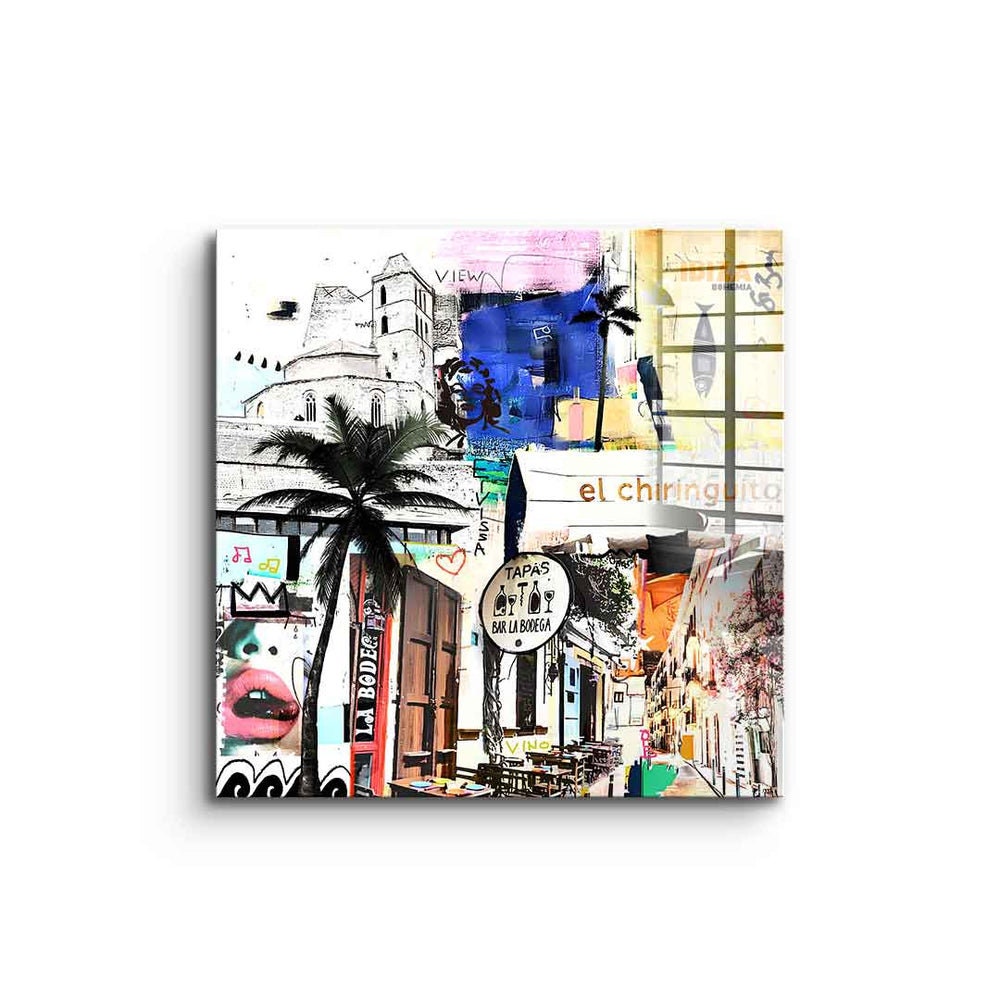The image is a detailed, conceptual wall hanging being sold on a site where digital imagery is transferred onto canvas. It features a chaotic montage of various scenes and objects. On the left side of the painting, there is a prominent palm tree, behind which appears to be a city wall adorned with graffiti, including lips, a crown, and music notes. The upper left corner showcases a black-and-white sketch of an old, fort-like building. Moving towards the center, the imagery transitions to an outdoor cafe with tables, surrounded by city streets and buildings, one of which bears a sign that reads "Taps" and displays bottles, indicating a tapas bar. The right side of the piece features an island-like scene at the top, and further down, additional city streets. In the middle of the composition, blue splashes interspersed with palm trees stand out. The color palette includes blues, light pinks (notably used for the lips), blacks, whites, browns, greens, oranges, and a pale yellow. The painting is a square-shaped montage that captures the essence of an eclectic urban environment with a mix of realistic and abstract elements.